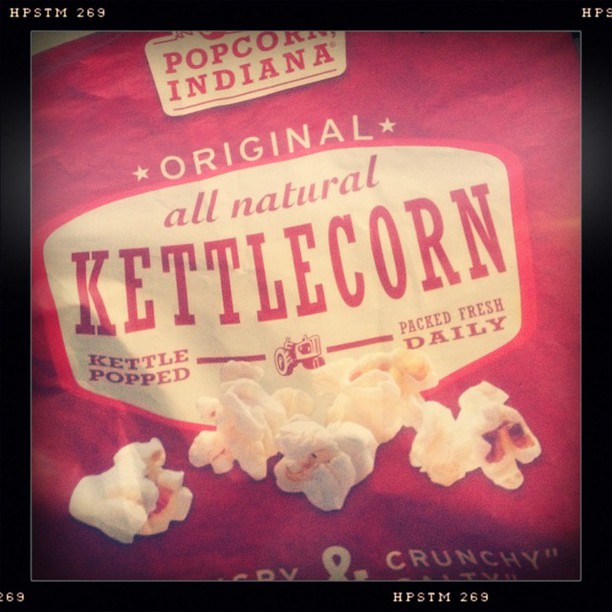This square image showcases the front of a vibrant red bag of Popcorn Indiana's all-natural kettle corn. The photo appears to be filtered with a popular Instagram sepia effect, giving it a warm vintage feel and framed with a black border, marked HPSTM 269. Inside the beige rectangle at the top, "Popcorn Indiana" is written in bold red letters. Below, another beige label with bulging top and bottom edges prominently displays "kettle corn" in large, white letters, with "all natural" above it in smaller text. The logo also features a small clip art image of a tractor, under which the words "kettle popped, packed fresh daily," are inscribed. Scattered at the bottom of the bag are about three to seven lifelike popped popcorn pieces, almost ready to be picked off. Additional text appears but is cut off; part of it includes the word "crunchy" surrounded by parentheses. The light crinkling of the bag adds to the tactile realism of the close-up capture.